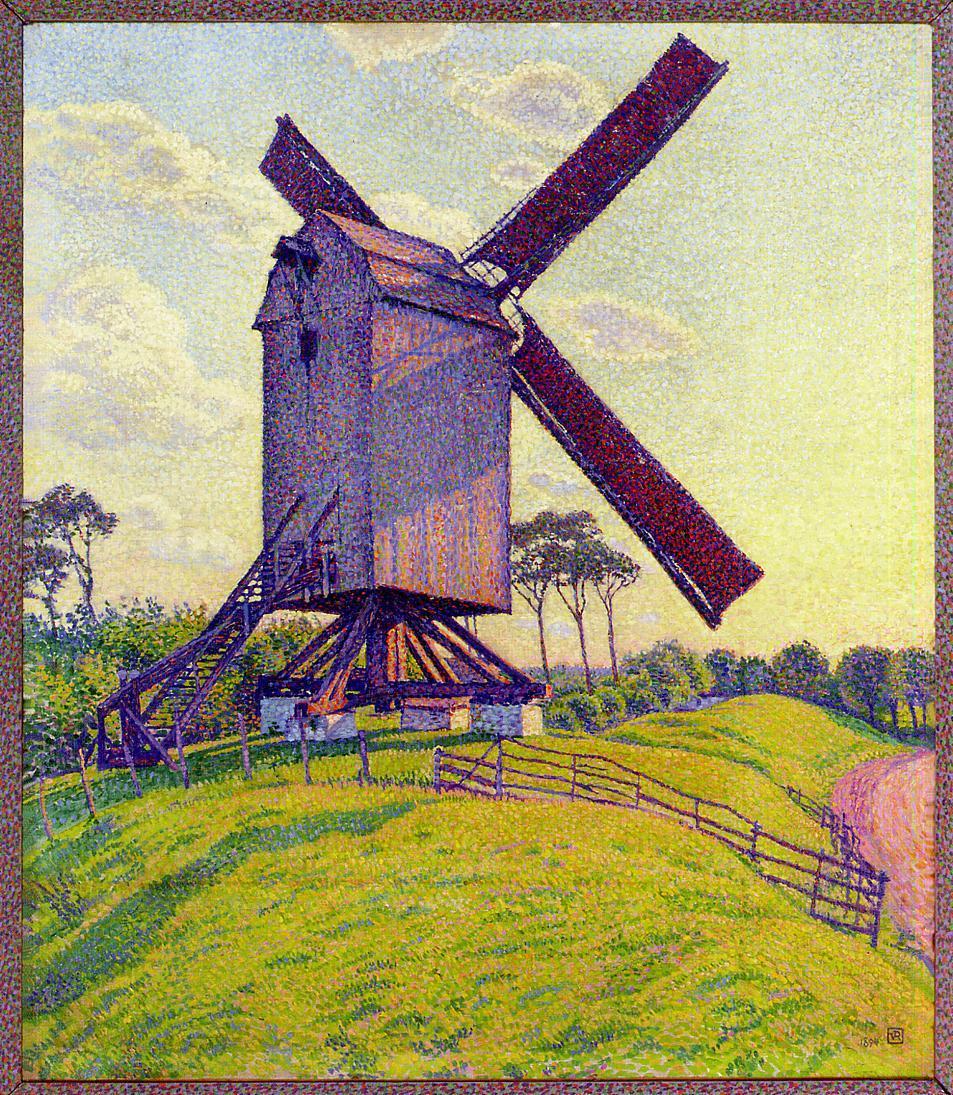This is a large vertical rectangular painting depicting an old windmill atop a green hill. The windmill, facing away from the viewer, is elevated on wooden stilts supported by white brick bases, which form a triangular structure leading up to the rectangular body of the windmill. The structure itself is brownish and appears to be wooden, with a triangular roof and a set of wooden stairs at the back. Three red wooden blades are visible protruding from the windmill. The scene is enclosed by a brown wooden rail fence, with a dirt road visible on the far right. The background features tall trees on either side of the windmill against a hazy, light blue sky dotted with white fluffy clouds. The hill is speckled with red accents, adding a vibrant touch to the landscape.